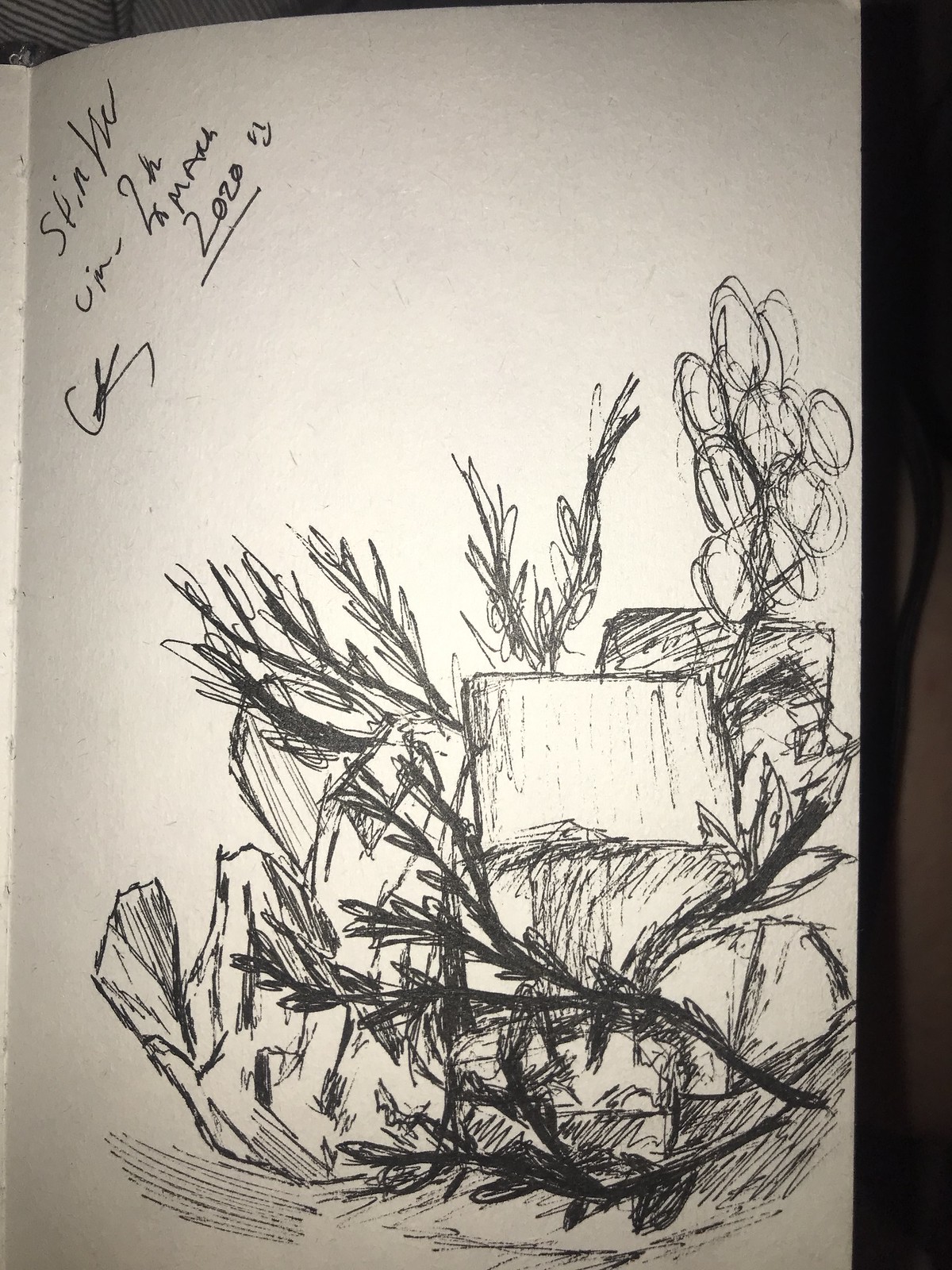This black-and-white photograph showcases a sketchbook opened to a page featuring an intricate still life drawing. The sketch appears to be rendered in ballpoint ink or possibly calligraphy pen on white paper. The left side of the image reveals a crease, indicating the spine of the book where the pages are bound together. The detailed still life includes a variety of natural elements such as sprigs of herbs with delicate leaves, several logs or branches, and clusters of berries or grapes on a stem. The artwork is signed in the upper left corner, along with the date "2020," attesting to its creation. The composition elegantly captures the textures and forms of these organic objects, giving a glimpse into the artist's observational skill and attention to detail.